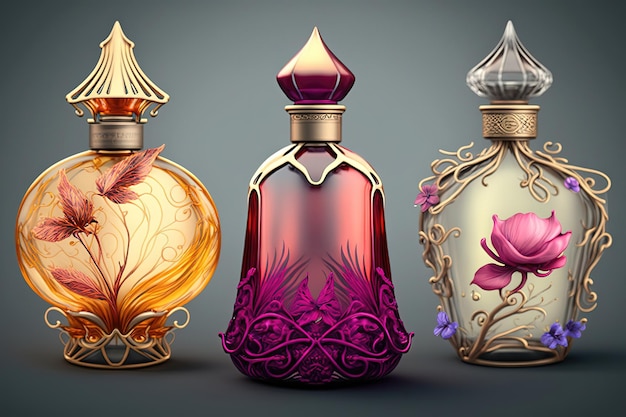The image depicts an array of three intricately designed glass perfume bottles, each adorned with elaborate decorations and ornate tops. The bottle on the left features an amber hue with orange flowers intricately carved into its rounded base. It boasts gold carvings around its base and a pointed, gold cap. The middle bottle, predominantly purple with gold trimming, has a cylindrical shape that is broader at the bottom and tapers slightly towards the top. It features fuchsia-colored, plant-like designs near the bottom, complemented by gold embellishments near the top, and is topped with a pointed, gold cap. The bottle on the right, characterized by its clear glass adorned with pink roses and purple-flowered carvings, is also embellished with botanical gold carvings resembling plant branches. Its transparent glass top completes its elegant appearance. Set against a gray background, these intricately decorated bottles stand out as the central elements of the image, each with distinct color schemes and detailed floral motifs that include flowers and butterflies, enhanced by delicate gold trimmings and ornate, pointed caps.